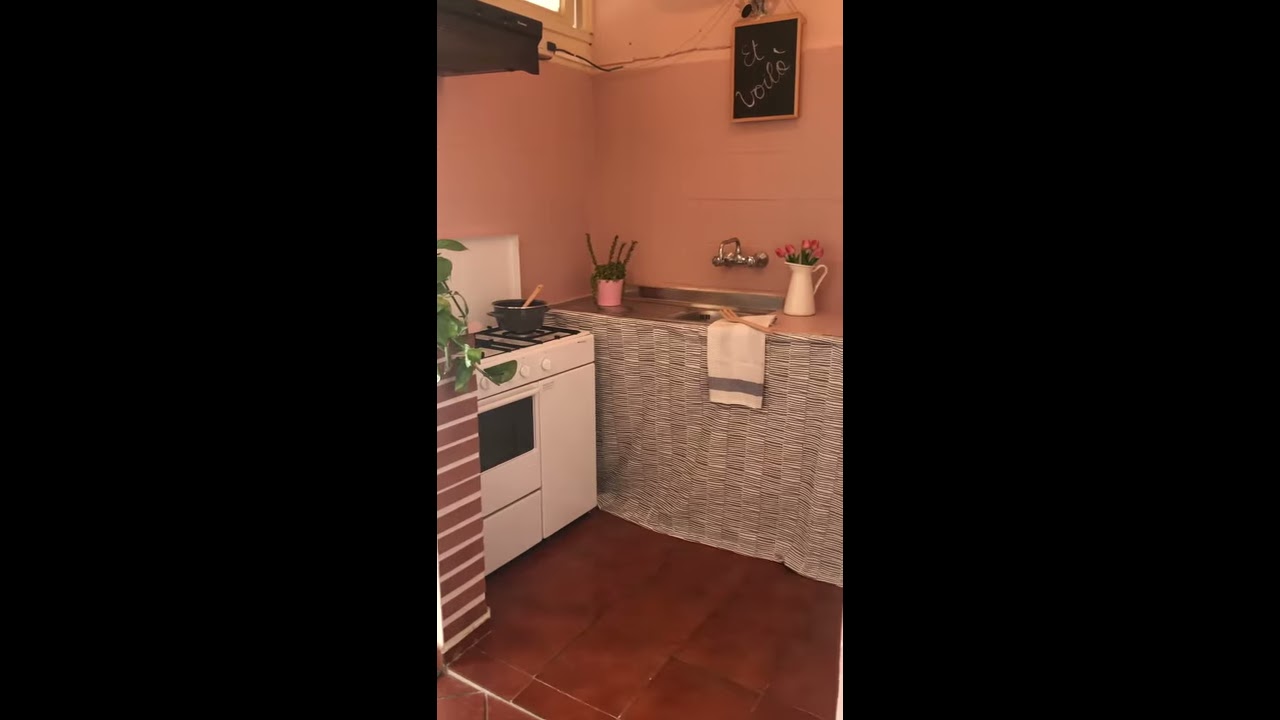This image showcases a small, meticulously clean kitchen. The kitchen has a compact layout with a white stove featuring two burners and a half oven, topped with a black pot and a wooden spoon. Adjacent to the stove, there's a stainless steel sink surrounded by a white and gray striped dish towel and a pink cup holding utensils such as a spatula and wooden spoon. A white vase filled with pink flowers adds a touch of color to the scene.

The kitchen floor is made of dark brown, stone-like tile with white grout, and the back walls are painted a light pink or peach color, creating a warm ambiance. The left side of the kitchen features red bricks with white concrete in between, giving a rustic feel. A chalkboard, possibly in Spanish, adds a decorative touch but is partly unreadable. 

To the left, a divider with brown and white horizontal stripes separates the kitchen from the next room, topped with the vibrant leaves of a pothos plant. There's a wicker curtain running off the countertop, likely hiding additional kitchen items. The overall space measures approximately 12 by 12 feet and is devoid of any active cooking, making it look picture-perfect and ready for future meal preparations.